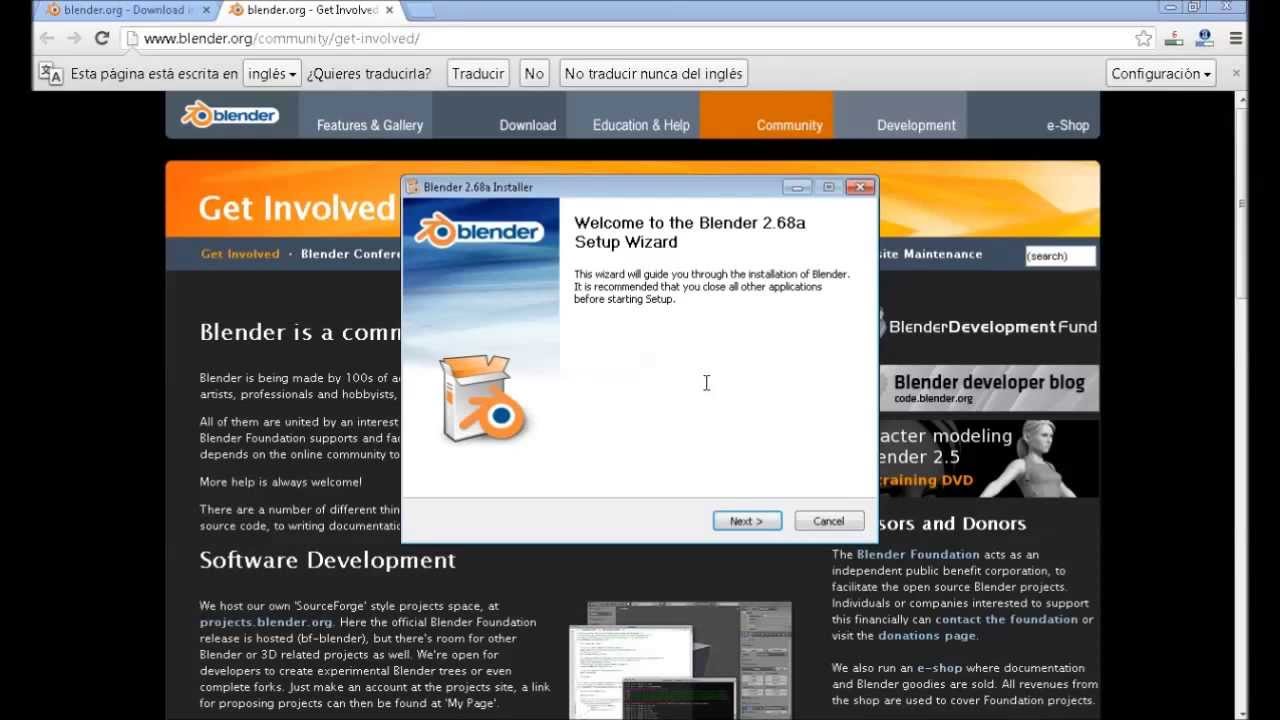This image showcases a detailed view of a website displayed within an Internet browser that features black borders. At the very top, there is a blue bar running horizontally with the text "blender.org-download" in blue letters. Next to this text, on the same tab, there is an 'X' indicating the option to close the tab. Adjacent to it, another tab is highlighted in gray, displaying "blender.org-getinvolved," also with an 'X' beside it.

Below the tabs, the browser interface includes standard navigation buttons—back and forward arrows, a refresh button, and an address bar containing the URL "www.blender.org/community/getinvolved." To the right of the address bar, there is a star icon for bookmarking the page, followed by additional menus or icons.

The next row features a drop-down box currently set to "inglés," next to Spanish text "esta página está escrita en," with more buttons and a "configuración" option positioned on the right side.

On the webpage itself, the word "blender" with an accompanying orange logo is prominently displayed. A horizontal menu bar below this includes various options: "features," "gallery," "download," "education and help," "community" (highlighted in orange), "development," and "eShop," with most options in shades of gray except for "community."

Beneath this menu, an orange row labeled "getinvolved" is visible. Additionally, a pop-up window overlaying the webpage details the "Blender 2.68a installer," featuring the Blender logo, and states "Welcome to the Blender 2.68a setup wizard," indicating that an installation process for Blender software is in progress.